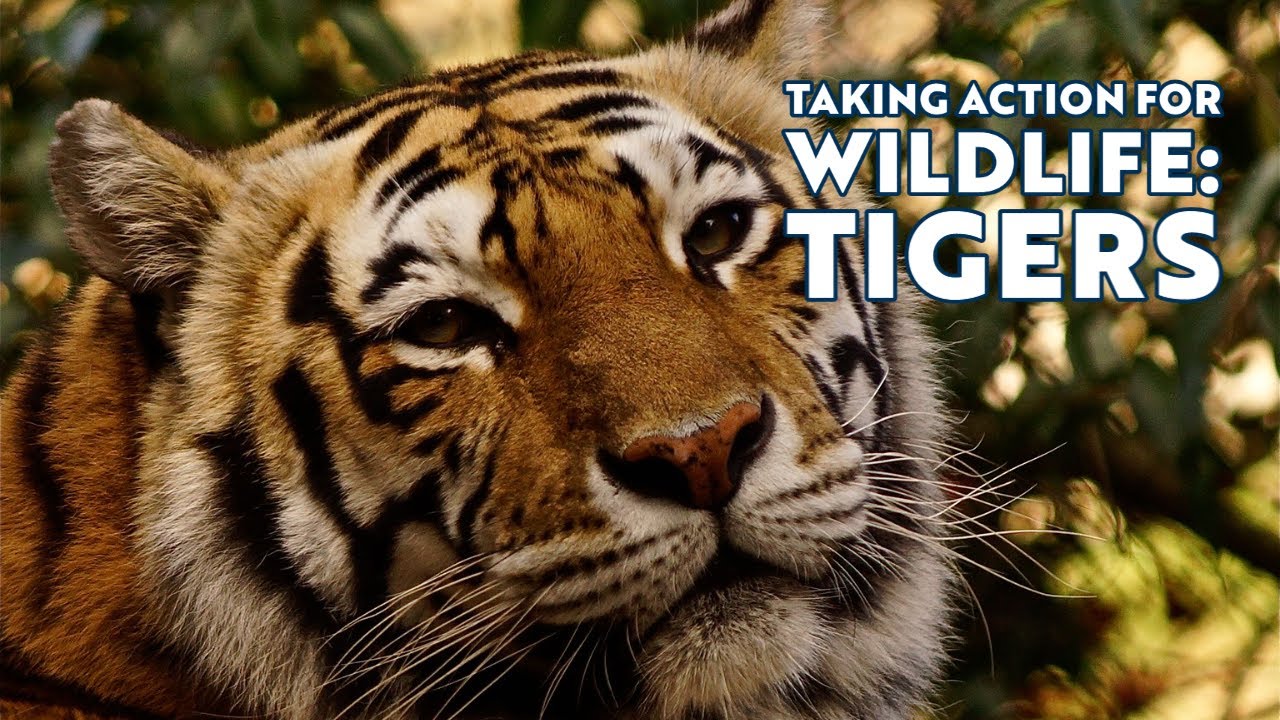The image features a close-up of a tiger's face with its head slightly tilted to the side, gazing calmly at the camera with partially closed eyes. The tiger displays the characteristic black, orange, and white coloration, with visible whiskers and ears, while its surrounding body remains out of the frame. Behind the tiger, a blurred green background suggests a natural outdoor setting. The top right section of the image features white text outlined in dark green, reading "Taking Action for Wildlife Tigers."